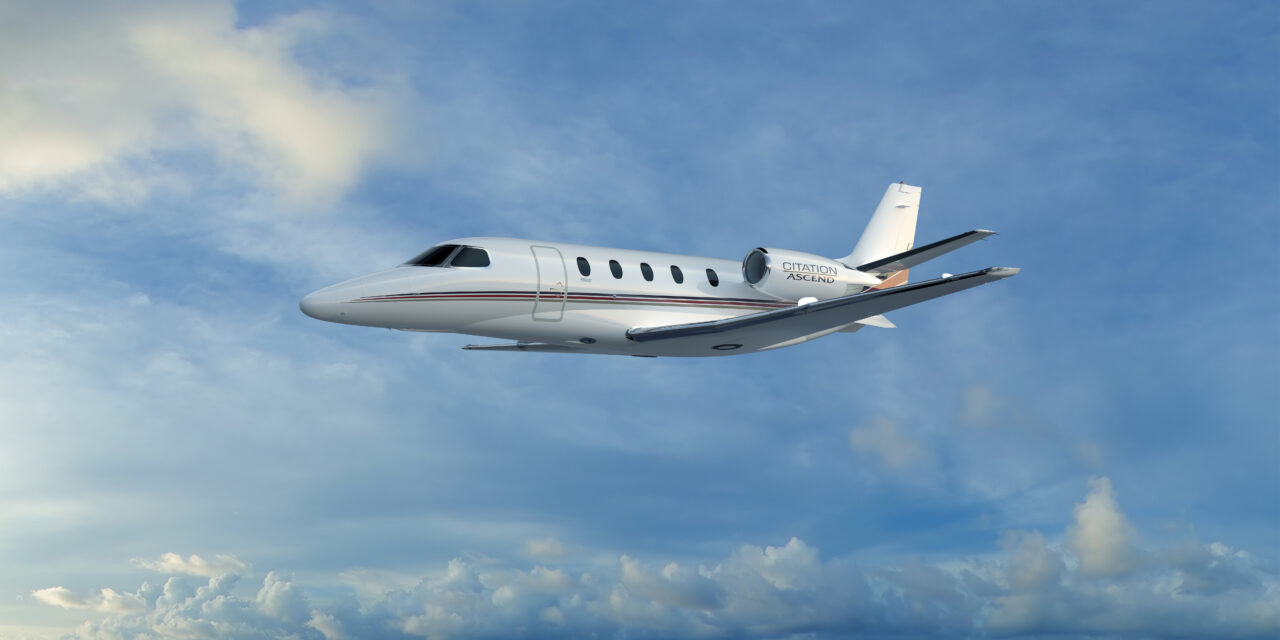The image depicts a small, private white jet airplane labeled "Citation Ascend" on the left engine, the text written in black. The jet is en route in a clear blue sky adorned with a few light clouds. The aircraft features five black-tinted windows on its side and a silver-framed door. Running from nose to tail, dark blue, red, and brown lines add a splash of color to the otherwise white fuselage. The plane is captured flying from left to right, with the tail on the right side of the image, highlighting the streamlined design and sleek appearance of the jet.